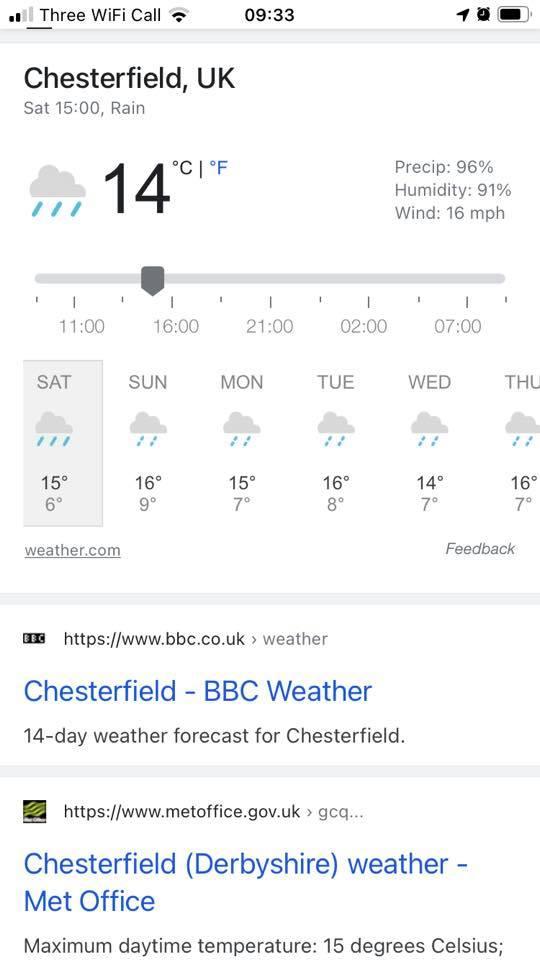A mobile screenshot displaying the weather forecast for Chesterfield, UK, in a vertical layout. The device uses 3 Wi-Fi call as its provider, and it's currently Saturday at 15:00 hours. The weather graphic indicates it's raining, with a temperature of 14 degrees Celsius. The interface allows selection of daily forecasts for the upcoming week, from Monday through Thursday, and possibly different timeframes for detailed weather predictions. Included in the details are expected highs and lows in Celsius, with significant rainfall forecasted. Below the main weather graphic, there are two search result links — one for Chesterfield’s BBC weather and another for Chesterfield Derbyshire Weather from the Metropolitan Office at office.gov.uk, providing additional sources to verify the weather information.